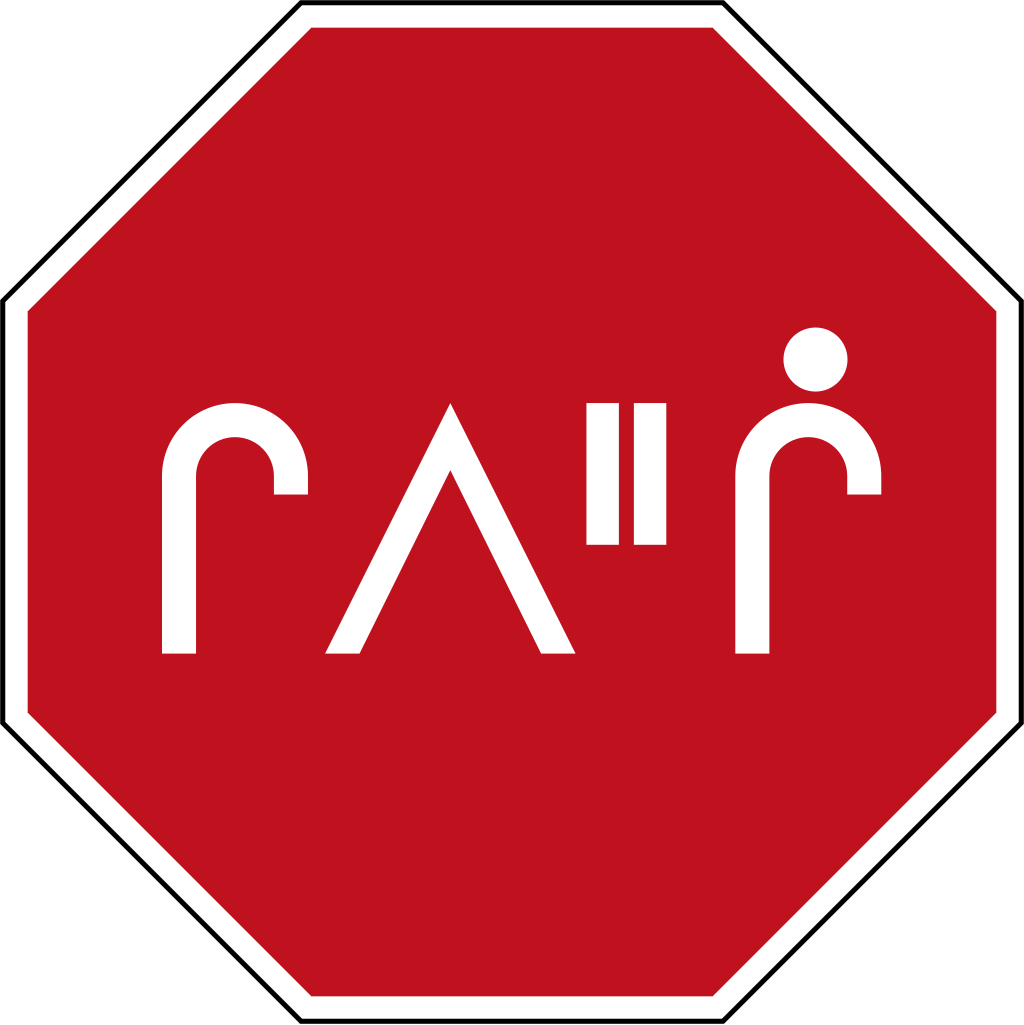The image is a computer-generated clipart of a stop sign. The sign is a classic red octagon with a thin white border around it, and an even thinner black outline surrounding the entire shape. Instead of the word "STOP," the center of the octagon features four symbols. The first symbol resembles a candy cane or a backward 'R', entirely white in color. The second symbol next to it is an upside-down 'V' or a triangle missing its base, depicted in white. The third symbol is a vertically oriented pair of white rectangles, akin to an equal sign rotated 90 degrees, and is about half the height of the other symbols. The fourth symbol is another candy cane shape, similar to the first, but with a small white circle above its arch, reminiscent of a lowercase 'i' dot.